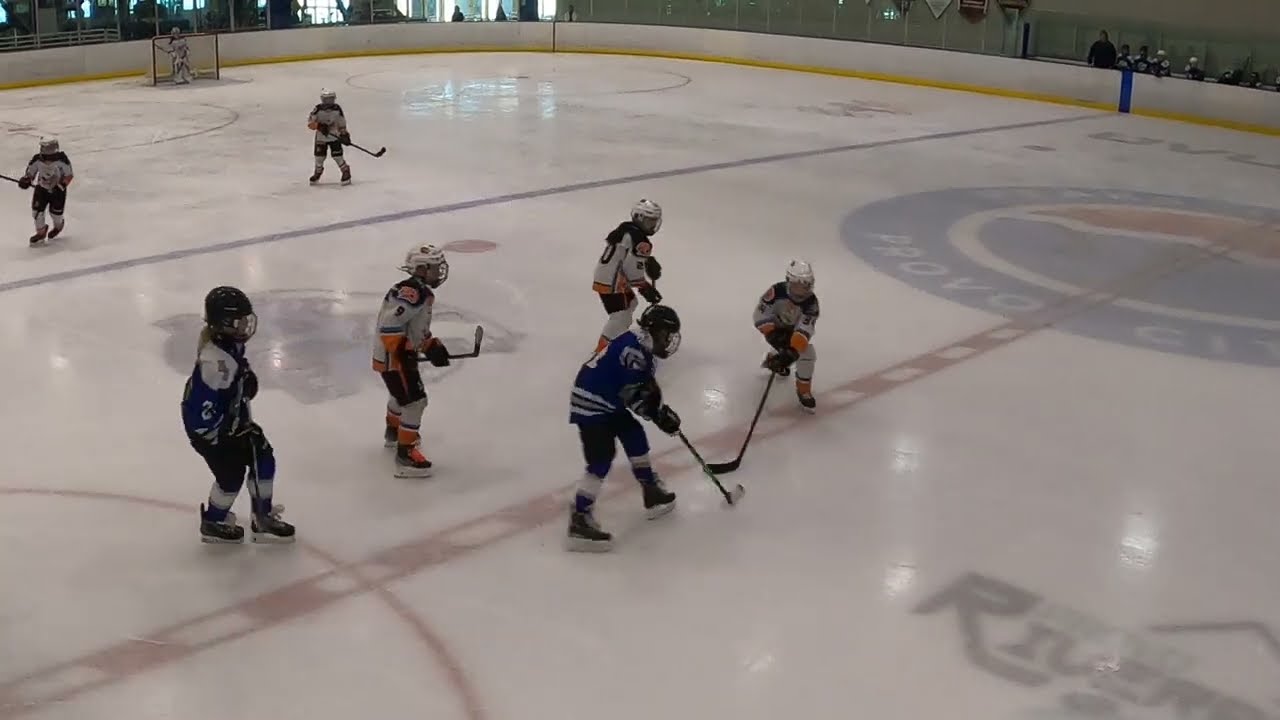The photograph captures an intense moment in a youth ice hockey game on a rink in Provo City, Utah. On the ice, there are eight young players actively engaged in the game. The white team, consisting of five players in white jerseys with yellow accents, has its goalie positioned near the net on the far left side. In the center of the rink, three of these white jersey players are closely interacting with two opposing players in blue jerseys. A puck is situated between one player from the blue team and one from the white, with additional players from both sides converging around them. The arena, featuring the Provo City logo in a blue circle at the center of the ice, exhibits dim lighting, casting a somewhat muted ambiance over the scene. To the upper right, a small number of spectators in the stands observe the competitive match.